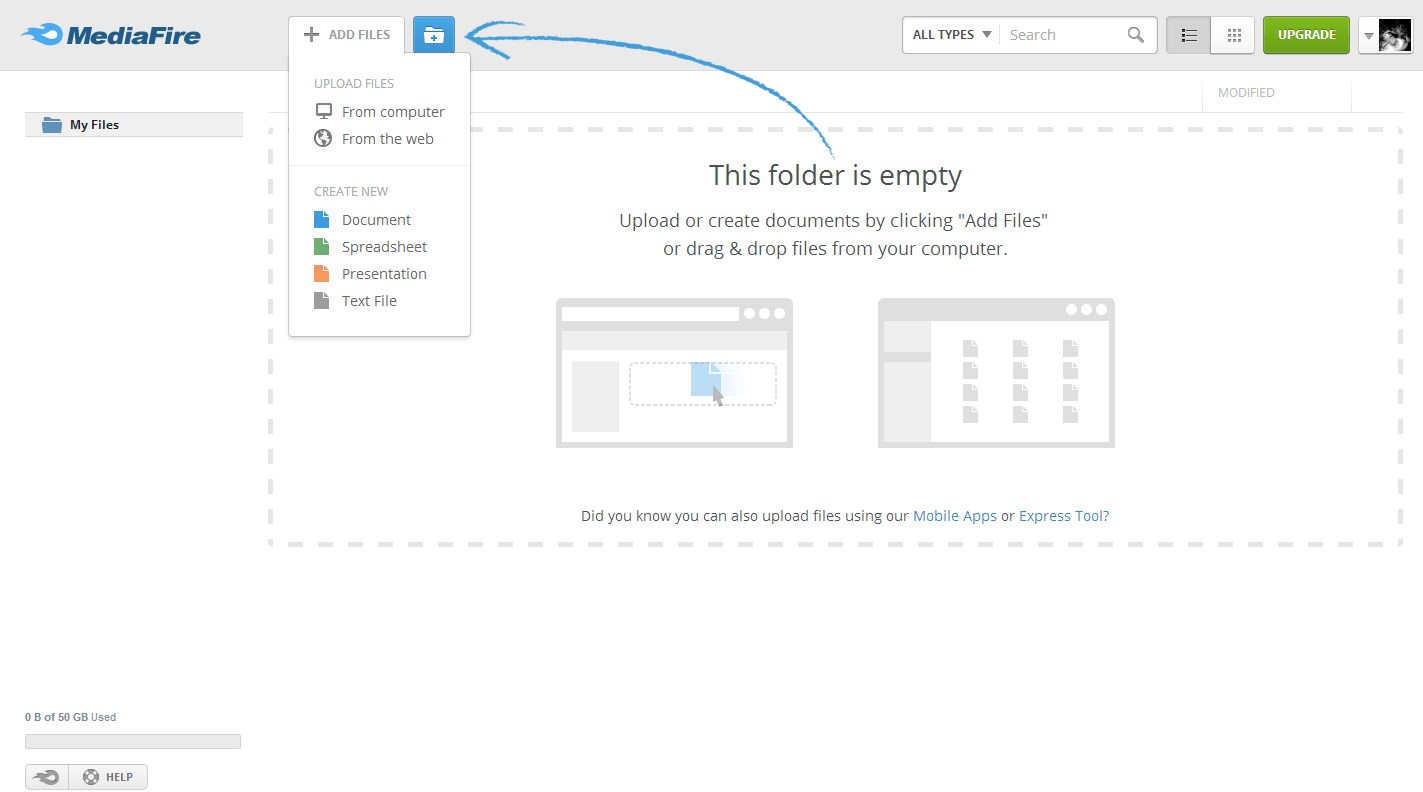Here is the revised and detailed caption:

A screenshot of a file management interface on a white background. At the top, there is a search bar labeled "All types" with a magnifying glass icon to the right. Adjacent to this, a green rectangle button labeled "Upgrade" is prominently displayed. Below, various sections and buttons are visible: "MediaFire" in blue, "My Files" in black next to a blue file folder icon, and a gray "Add Files" button with a gray plus sign. The interface offers options to upload files with labels such as "From Computer," "From the Web," and "Create New." Under "Create New," options include "Document" represented by a blue sheet of paper, "Spreadsheet" with a green sheet of paper, "Presentation" with an orange sheet of paper, and "Text File" illustrated by a gray sheet of paper.

At the center of the screenshot, a large blue square contains a white file folder icon with a message indicating, "This folder is empty." A blue arrow points to this blue square with the file folder icon. An instructional message states, "Upload or create documents by clicking 'Add Files' or drag and drop files from your computer." Additional notes include, "Did you know you can also upload files using our mobile apps," and "Express 2," both in blue text for emphasis. In the bottom left corner, the usage bar shows "0B of 5.0 GB used."